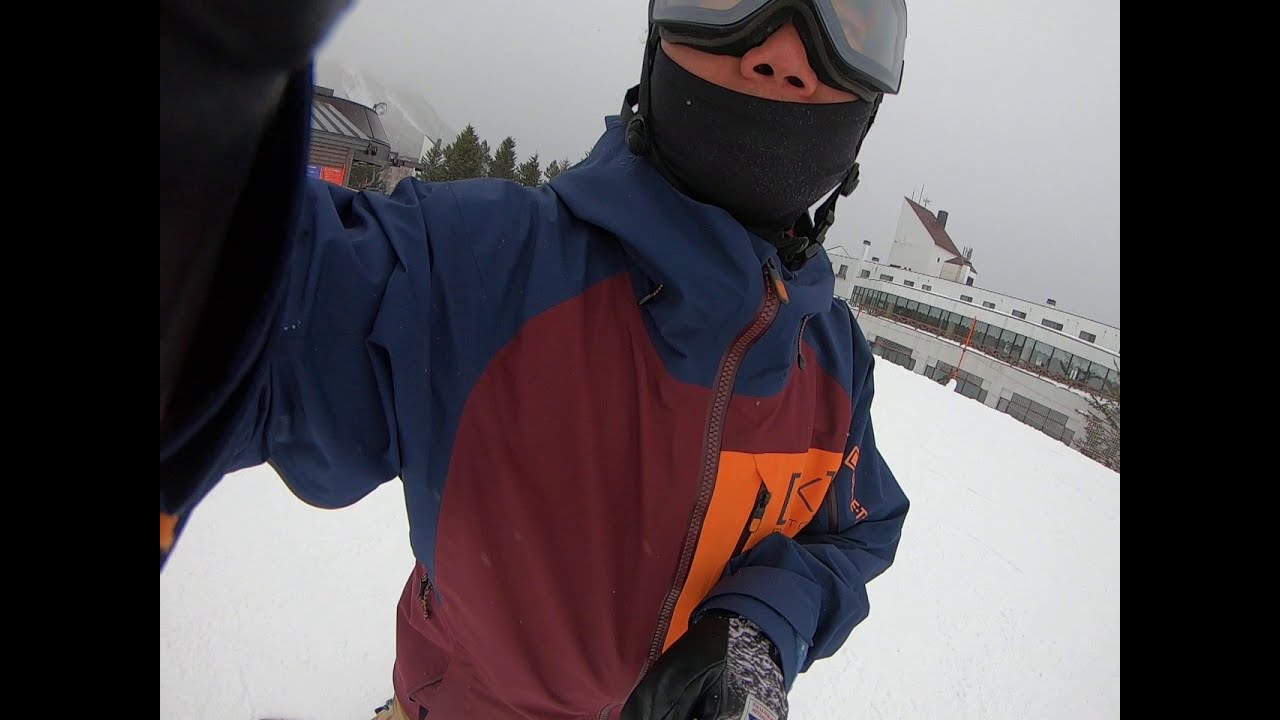In this image, a man, centrally positioned, takes a selfie while standing on a snow-covered hill, dressed in full ski gear including black-lined goggles, a black balaclava, a multi-colored windbreaker with blue sleeves, and red and orange in the center, and black ski gloves. His right hand is extended outward, holding the camera towards himself, while his left hand rests at his waist. The ground around him is blanketed in snow, suggesting a thick layer, as evidenced by a pole in the background sticking up through the snow.

The setting appears to be a cold, wintery, mountainous outdoor area, possibly a ski slope midday. The sky is predominantly foggy, maybe due to cold weather or an approaching storm. In the background, on the left side, faintly visible, are some evergreen trees, a small building, and a mountain with a ski trail. On the right side of the image, there is a large multi-story brick building with numerous glass windows, potentially a lodge or complex, and farther back, a snowy mountain peak. This scene captures the stark coldness and vastness of a skier’s high-altitude adventure.